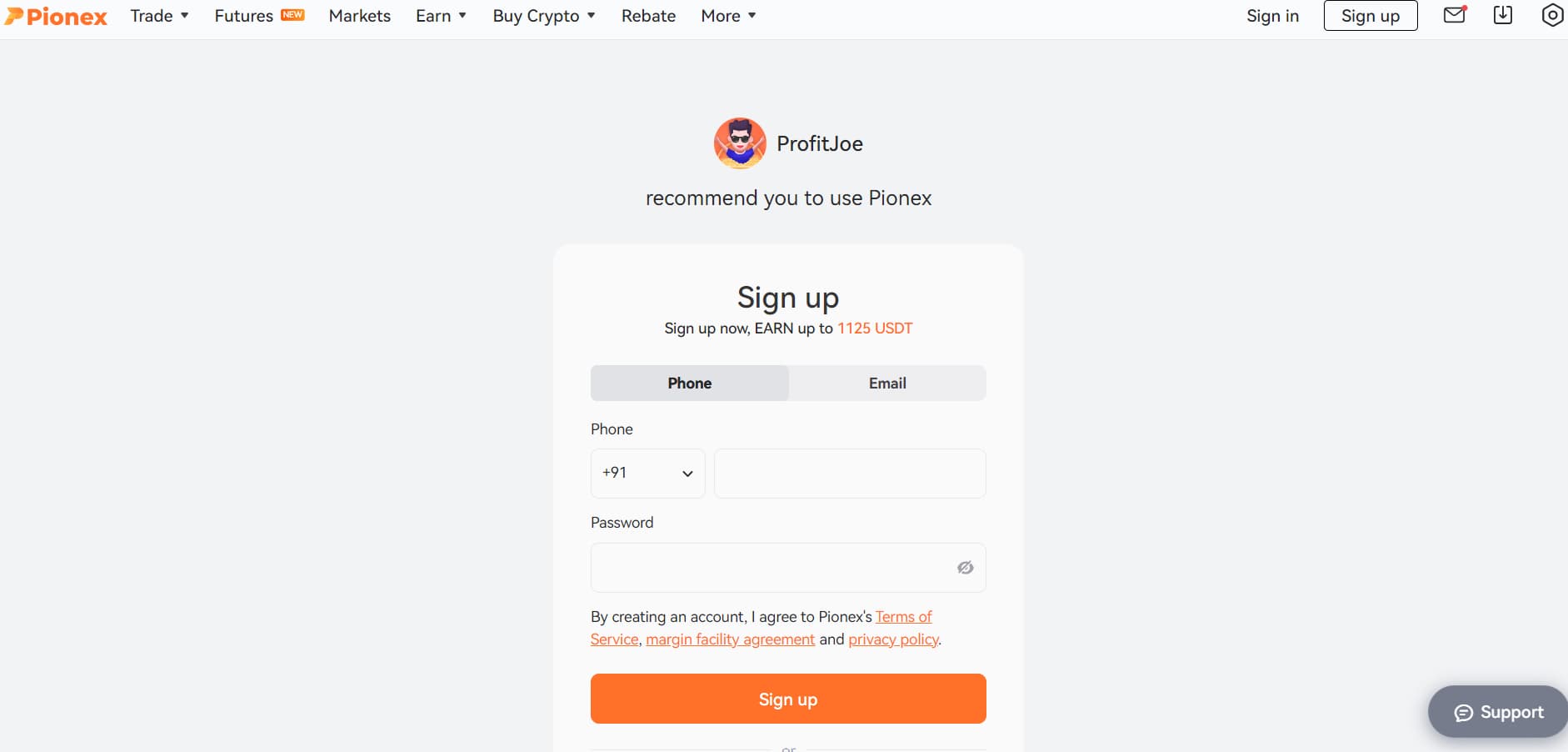The image depicts the homepage of the Pionex (PIO and EX) cryptocurrency trading platform, presented with a predominantly orange and white color scheme. On the left side, the site's logo, "Pionex," is highlighted in orange. A vertical navigation menu allows users to access various sections via pull-down menus, including "Trade," "Futures," "Markets," "Earn," "Buy Crypto," "Rebate," and more.

On the right side, there are options to "Sign In" and "Sign Up." An envelope icon with a red notification circle and an additional "Download" image and "Settings" icon are visible. The central part of the page prominently promotes an offer: "Profit Joe recommends you to use Pionex (PIO and EX). Sign up now and earn up to 1125 USDT." 

The sign-up form below features tabs for phone and email registration, with a placeholder for the international phone code "+91" and an input field for the phone number. The password field beside the eye icon has a slashed line indicating hidden text.

At the bottom of the form is a disclaimer: "By creating an account, I agree to Pionex's terms and services, margin family agreement, and privacy policies," with the relevant links underlined in orange. A conspicuous "Sign Up" button in orange with white text is present.

In the bottom right corner of the image, there is a "Support" option encased in a gray bubble with white text.